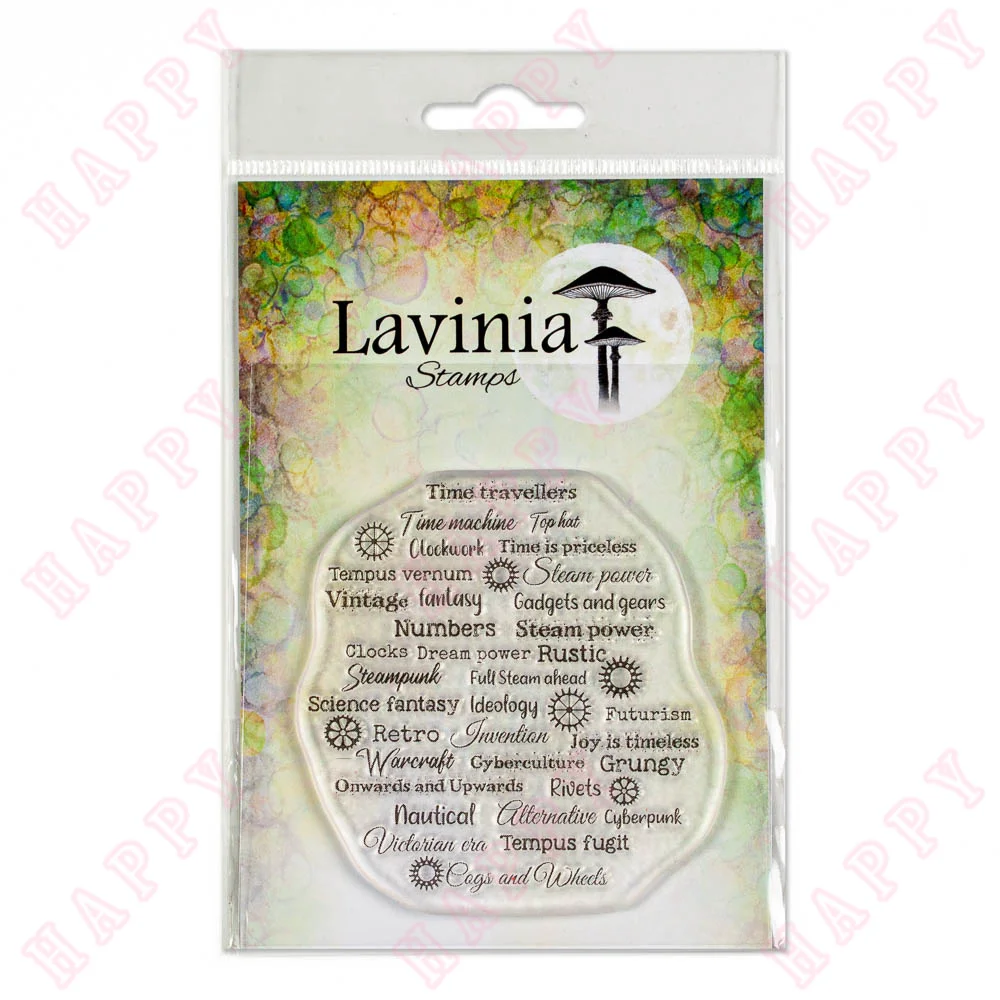This image features an intricate collection of themed stamps prominently arranged to catch the eye. The majority of the stamps bear significant words such as "Time Travelers," "Time Machine," "Futurism," "Ideology," "Retro," "Science Fantasy," and "Steampunk." These words suggest a cohesive theme centered around the concepts of time, imaginative futures, and speculative pasts, evoking genres like steampunk and science fiction. Interspersed among the word stamps are several that depict intricate cogs, rendered in dark hues of black and deep brown, adding a mechanical and industrial aesthetic to the collection.

The stamps are contained within a package branded with the name "Lavinia," clearly inscribed as "Lavinia Stamps." The branding features a distinctive logo that showcases an enchanting design: two mushrooms positioned against the backdrop of a moon. This whimsical logo enhances the fantasy and artisanal charm of the stamp collection.